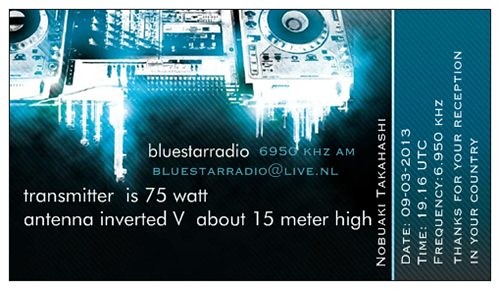The image is an advertisement for "Blue Star Radio" operating at 6.950 kHz AM. The left two-thirds of the image feature a black background with a central picture of DJ turntables and a mixer. Above the image, "Blue Star Radio" is written in bold white text alongside "6.950 kHz AM" in blue text. Below this, the email address "BlueStarRadio@live.nl" is displayed. Further down in white text, it reads: "Transmitter is 75 watt" and "Antenna inverted V, about 15 meters high." Vertically aligned along the left edge is the name "Nobuaki Takashi" in white font. The right third of the image has a blue background with white text providing details: "Date: 09-03-2013," "Time: 19:18 UTC," "Frequency: 6.950 kHz," and a note, "Thanks for your reception in your country." The advertisement effectively showcases the radio station's transmission details and contact information.